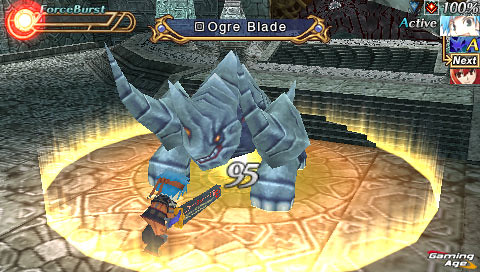The image is a detailed screenshot from a video game, likely a fighting game or RPG. At the center, a massive bluish-gray monster resembling a rhinoceros stands menacingly. The creature is characterized by its stony or metallic texture, a prominent horn, sharp teeth, and glowing angry orange eyes. Surrounding the monster is a large ring of orange magical light, further amplifying its intimidating presence. 

In front of the beast, a player character engages from a close distance, armed with a giant chainsaw. The character's specific features are obscured by the bright magical effects, but other descriptions indicate they might be wearing a brown and black suit, with blue hair and a red bandana. This standoff takes place within a castle-like environment, evident from the stone stairs and platform visible in the background.

Above the monster is a blue banner bearing the text "Ogre Blade" in white. Additional game interface elements are scattered across the screen: an energy meter labeled "Force Burst" in the upper right corner, a status marked "Active, 100%," a "Next" prompt, and various game icons. The number "95" is displayed prominently near the creature, likely indicating its level or health. The whole scene may include subscriptions or branding elements like "Gaming Age" at the bottom right.